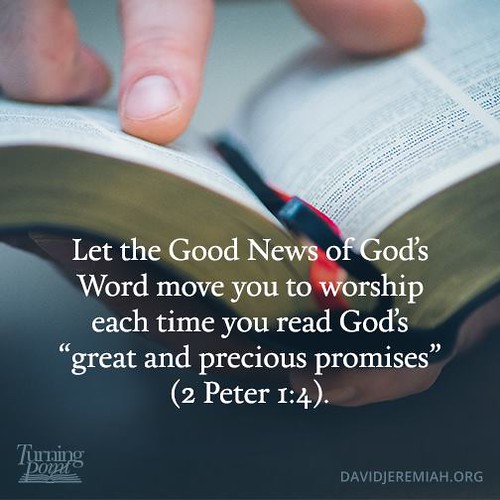The image portrays an open book, likely a Bible given its appearance and context. The book's pages are white, filled with dense, illegible black text, and its cover is black, seen only partially due to the angle. A hand, coming from the top left, holds the book open, with the index finger pointing to a specific spot. Superimposed in white font over the photograph is the Bible verse: "Let the good news of God's word move you to worship each time you read God's great and precious promises," from 2 Peter 1:4. Additionally, on the bottom left, there's a logo featuring the text "Turning Point" accompanied by a graphic side view of an open book. The bottom right corner displays the text "davidjeremiah.org." The image employs a mix of tan, pink, black, white, brown, and gray hues, emphasizing a motivational, church-related theme centered around the uplifting message of the verse.